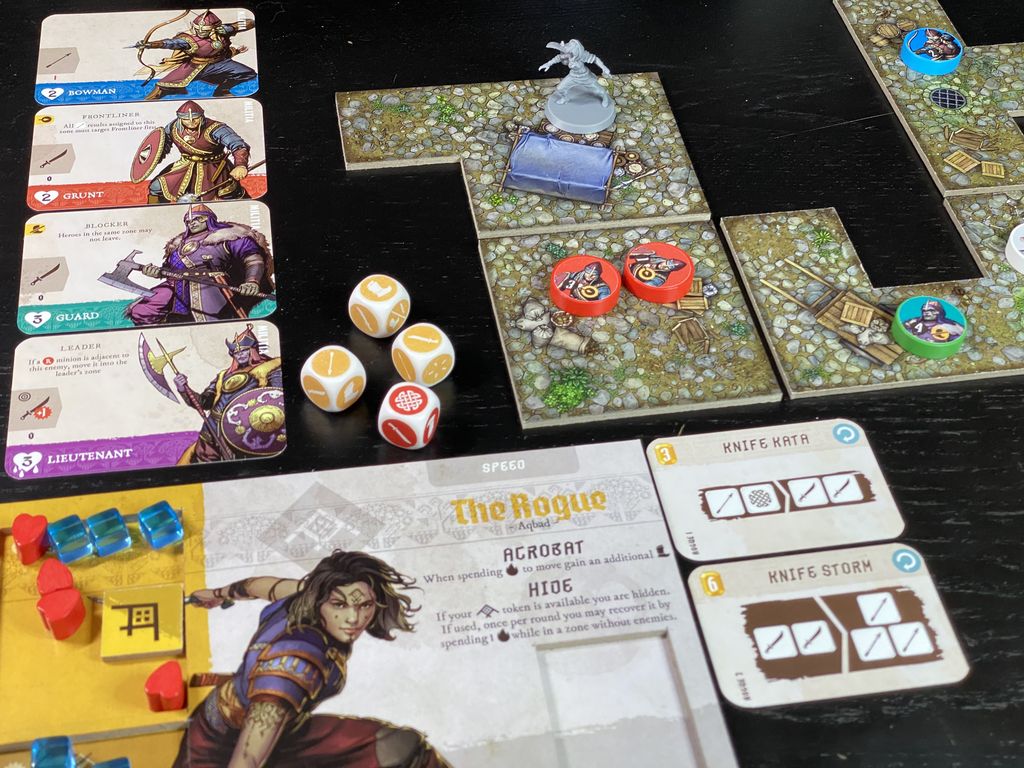This photograph captures a detailed setup of a role-playing board game, meticulously arranged on a dark wooden table, whose planks run horizontally across the image. The focal point is a game board in the upper right corner, resembling a stone-paved path for player movement. Scattered around the board are a variety of game pieces, including small circular icons and figurines resembling silver dragons and warriors.

Central to the arrangement are five dice, all white with distinctive markings: three feature yellow designs, while one showcases red designs. To the left of these dice are four index card-sized pieces of paper, each depicting a different warrior character. These cards have a white background with various colored borders—blue, orange, teal, and purple—each illustrating knights in medieval-style armor with various weapons like bows, axes, shields, and swords.

On the lower left, there is a collection of smaller game components, such as red heart-shaped tokens and blue square pieces, reminiscent of ice cubes. Among these, additional cards labeled "Knife Kata" and "Knife Storm" are visible. In the foreground lies the game box showcasing a young character in leather armor, poised for combat, with the game’s title, "The Rogue," prominently displayed. The box and other elements feature text in an unidentified language, adding an exotic touch to the game’s mystique.